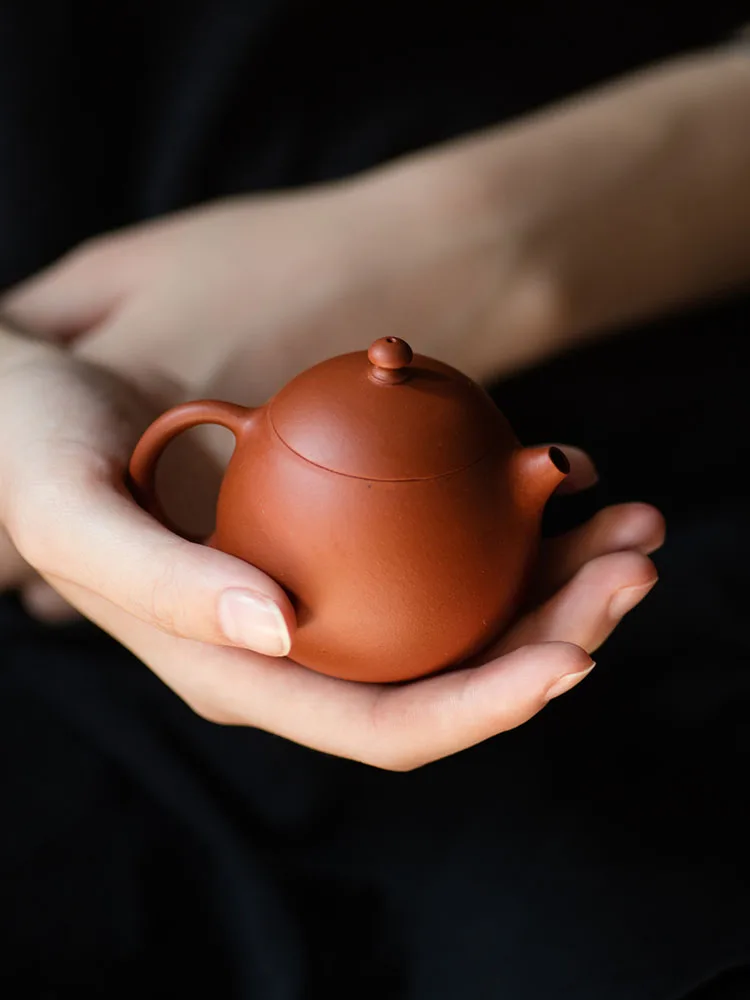In this professional-quality close-up image, we see a small, bronze-colored teapot cradled in the right hand of a woman dressed in black. The teapot is small enough to comfortably fit in the palm of her hand, and features a short spout and a simple, knob-topped lid. The reddish-brown teapot, with its matte but somewhat shiny finish, is clearly the focal point of the composition, contrasting against the blurred, black-clad background. The woman's left arm is visible resting at her waist, contributing to the symmetrical and balanced framing of the image. The meticulous focus on the teapot and the hand holding it accentuates the minimalist aesthetic and high-quality details of the photograph.